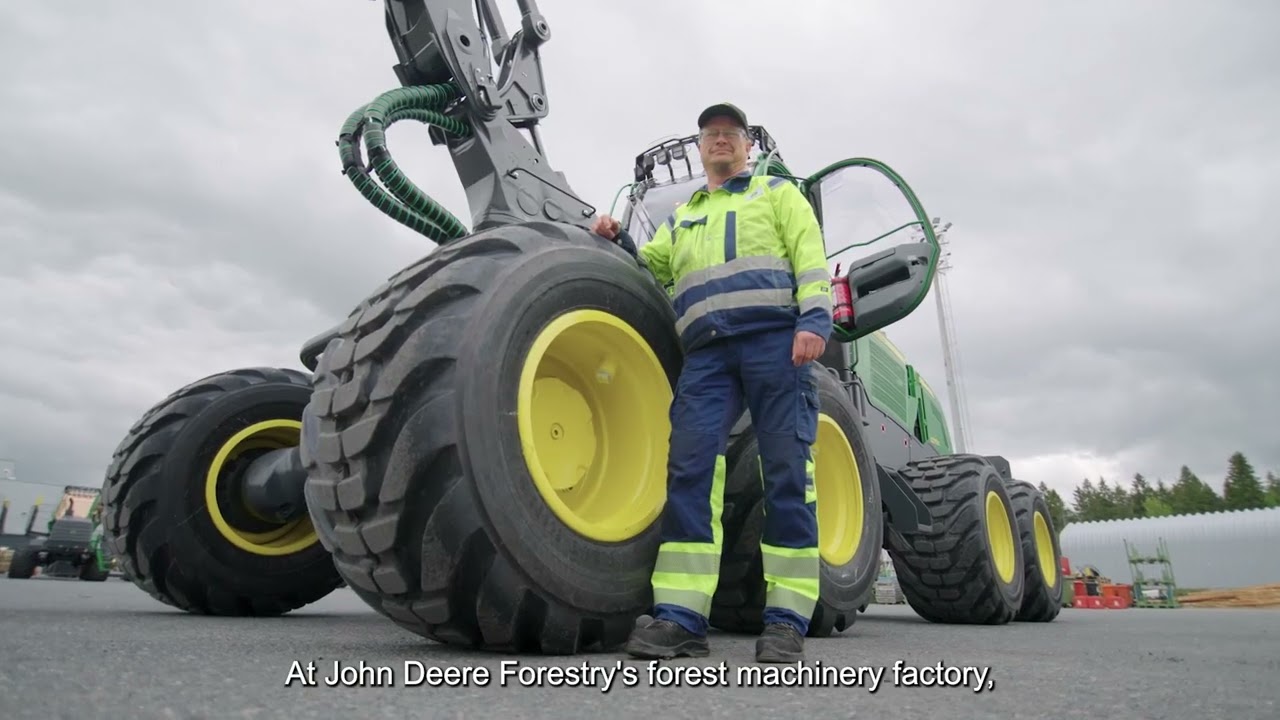In this image, you see a man dressed in safety attire standing beside an enormous piece of John Deere forestry machinery at the John Deere Forest Machinery Factory. The man is wearing safety glasses, a cap, and a neon yellow and blue jacket with reflective gray stripes, along with pants that have yellow-striped safety sections and sturdy safety shoes. The massive green tractor has eight large wheels with yellow inserts. The right side of the vehicle and its massive tires are prominently visible. The door to the operator’s cabin is open behind the man, revealing part of the inside. Extending from the tractor is a large hydraulically operated arm reaching towards the sky. In the background, you can see a fence, several trees, and a cloudy, gray sky, along with another John Deere tractor. The caption below the image reads, "at John Deere Forest Machinery Factory." The photograph is taken from a low angle, making the machinery appear even more colossal compared to the man. The scene is set on a paved surface.